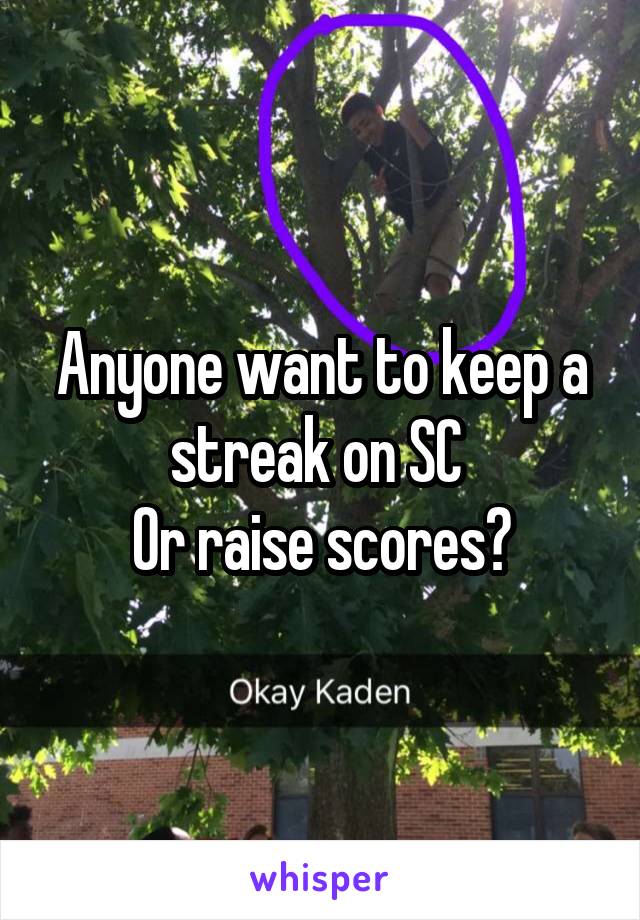This image appears to be a meme or social media post featuring a photograph taken outdoors. The focal point is a young boy, dressed in a navy or black shirt and brown shorts, who is climbing a tall, leafy tree. The boy is about halfway up, standing on one branch and holding onto another, with a brick building visible in the background and sunlight filtering through the leaves. The boy is circled in purple, highlighting his position in the tree. Overlaying the image in white text are the words, "Anyone want to keep a streak on SC or raise scores?" followed by "OK Caden" beneath it, which is written atop a black banner. At the very bottom of the image, written in purple against a white border, is the word "whisper." The colors in the image include various shades of green, brown, black, red, and purple. The overall setting and style suggest that this is intended to be shared on social media.